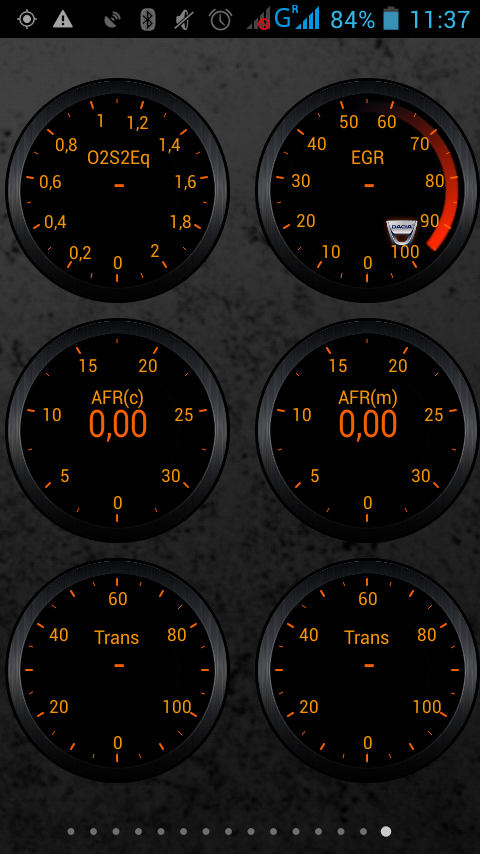This is a highly detailed screenshot of a smartphone display featuring six distinct dials against a black background. The top of the screen showcases standard smartphone icons from left to right: a circle, a triangle with an exclamation point, a sound icon, a squiggly symbol, a mute button, a clock icon, a red icon with a slash through it, the letters 'G' and 'R' in proximity, blue cellular signal bars indicating connectivity strength, and finally, the battery life displayed as '84%'. Adjacent to these icons, the time is indicated in blue as '11:37'.

The focal point of the image comprises six separate circular dials, each featuring various numeric readings including fractions and whole numbers. Despite their resemblance to clocks, these dials serve different functions. The top-left dial is labeled '02S2EQ' with numbers encircling it. The top-right dial is labeled ‘EGR’ and includes numbers as well as a striking red line. The middle row consists of two dials; the left one labeled 'AFR (C)' and the right one labeled 'AFR (M)'. Each dial presents a unique set of numbers. Finally, the bottom row displays two identical dials labeled 'trans', again surrounded by numerical data.